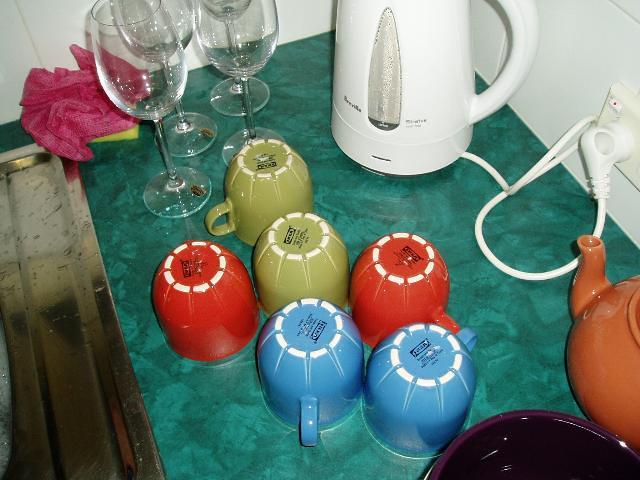The image depicts a kitchen counter or a dresser with a green laminate surface that has a flecked pattern. At the back right corner, there is a white electric kettle plugged into a wall socket, and it features a handle. The kettle is almost empty. In the center of the countertop, six teacups are positioned upside down for drying; they include two of each color: blue, red, and green with white rims and small black writing on the base. A purple bowl and an orange ceramic teapot with a visible spout occupy the lower right corner. At the upper left corner of the counter, three clean and shiny wine glasses stand upright beside a purple crumpled napkin. A sponge and dishcloth are also visible near the top left corner. The setup is against a solid white wall.